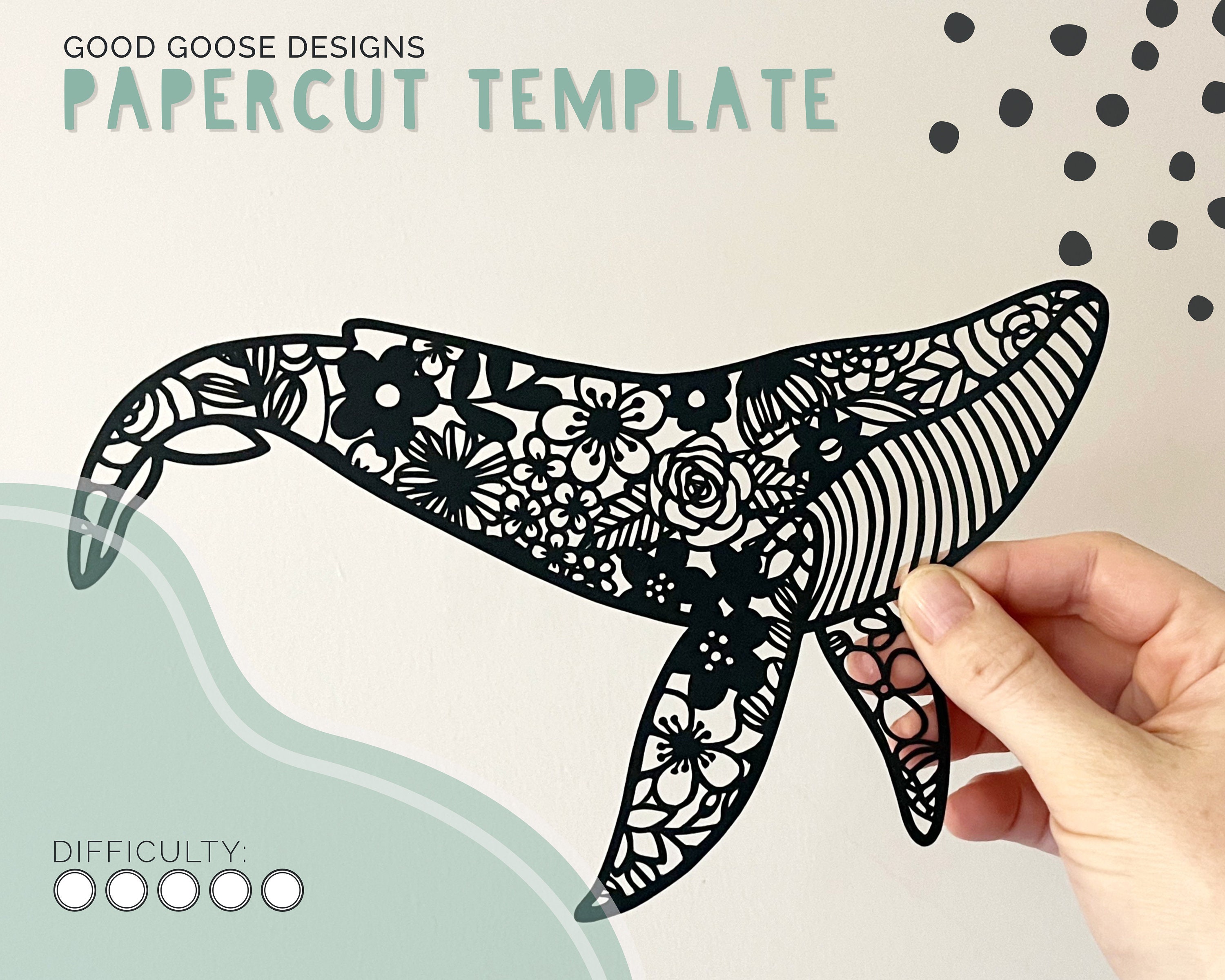The image features a close-up of a person's right hand holding a decorative, intricately designed template of a whale. The whale appears to be made of a metallic or plastic material and is adorned with a complex pattern of black flowers, leaves, and curved lines. The design is see-through with gaps allowing the background to be visible. 

At the top left corner in small black letters, the text reads "Good Goose Designs," and below it, in larger light blue letters, it says "Papercut Template." On the top right, there are several black circles against the light background. The whale is held by the hand near one of its flippers and below its chin, suggesting it could be emerging from the water, as indicated by the wavy line features at the bottom left of the image. 

Additionally, the bottom left corner displays the word "Difficulty" in black, followed by five white circles, likely indicating the complexity level of the template. The background in this area transitions into light blue wavy lines, enhancing the visual appeal of the design.